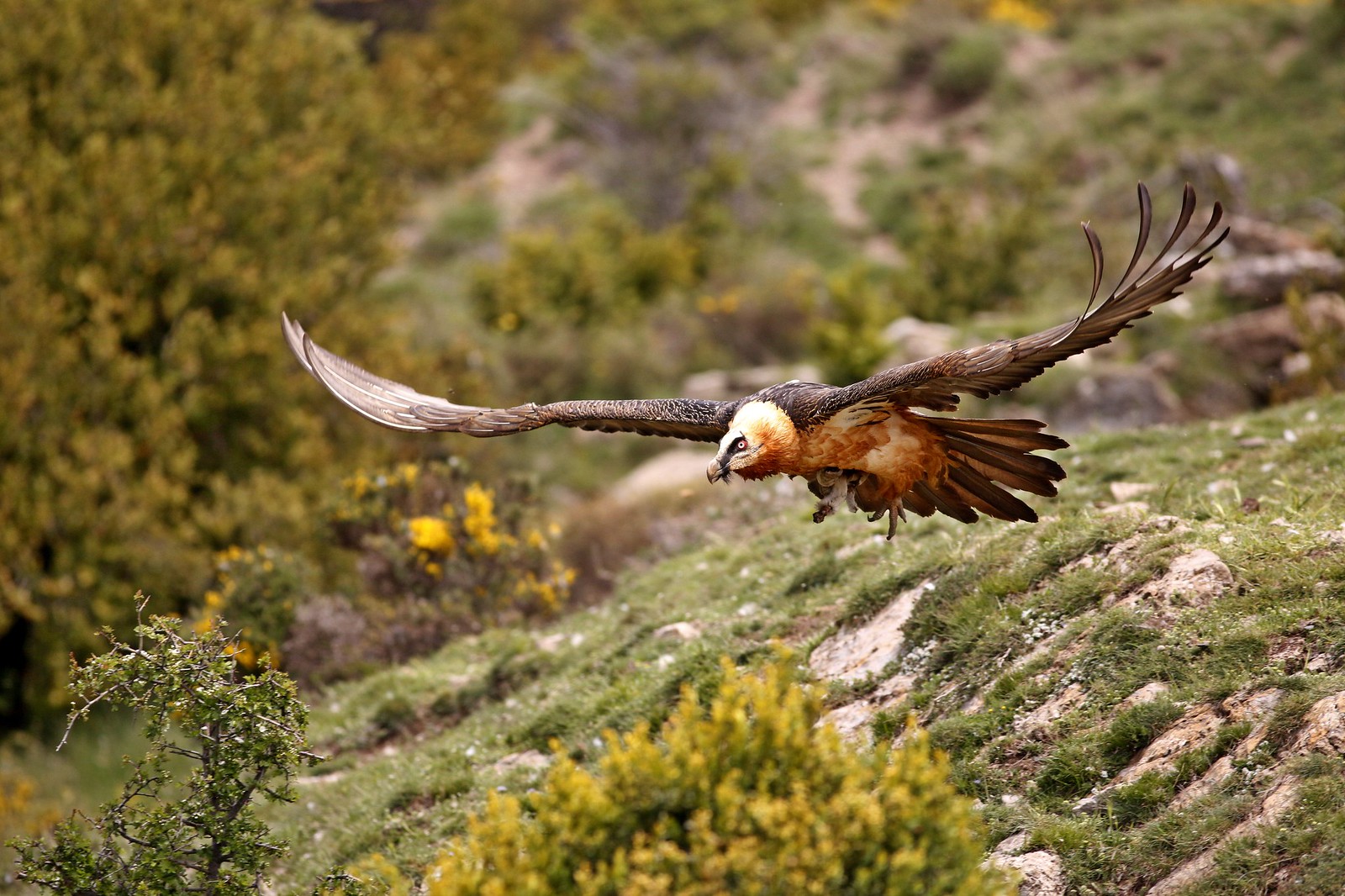In this outdoor daytime photograph, a white-headed vulture is captured in mid-flight, swooping from the right-hand side to the left. The bird, which is not a bald eagle, is prominently displayed with its long wings spread wide, revealing dark brown wing feathers with tips flaring outward and upward. The vulture's head is distinctly white, contrasting with its reddish-brown body, which features lighter brown and orangish tones on the abdomen and neck. The bird's tail feathers are also dark brown and are spread out, while the claws of its left foot hang downward, and its right foot grips a small white furry animal close to its body. The vulture's beak transitions from light brown at the tip to black near the base, complementing its white iris and black-pupil eyes with reddish skin behind them. Below and behind the bird lies a rocky hillside dotted with bushes, shrubs, and smaller trees, all slightly out of focus, giving depth to the scene. Yellow flowers and tan dirt patches are also visible amidst the greenery, enhancing the natural setting. The photograph is right triangular in shape, being wider than it is tall, and places the bird's body just right of the centerline, with its wingspan extending about three-fourths of the way across the image.